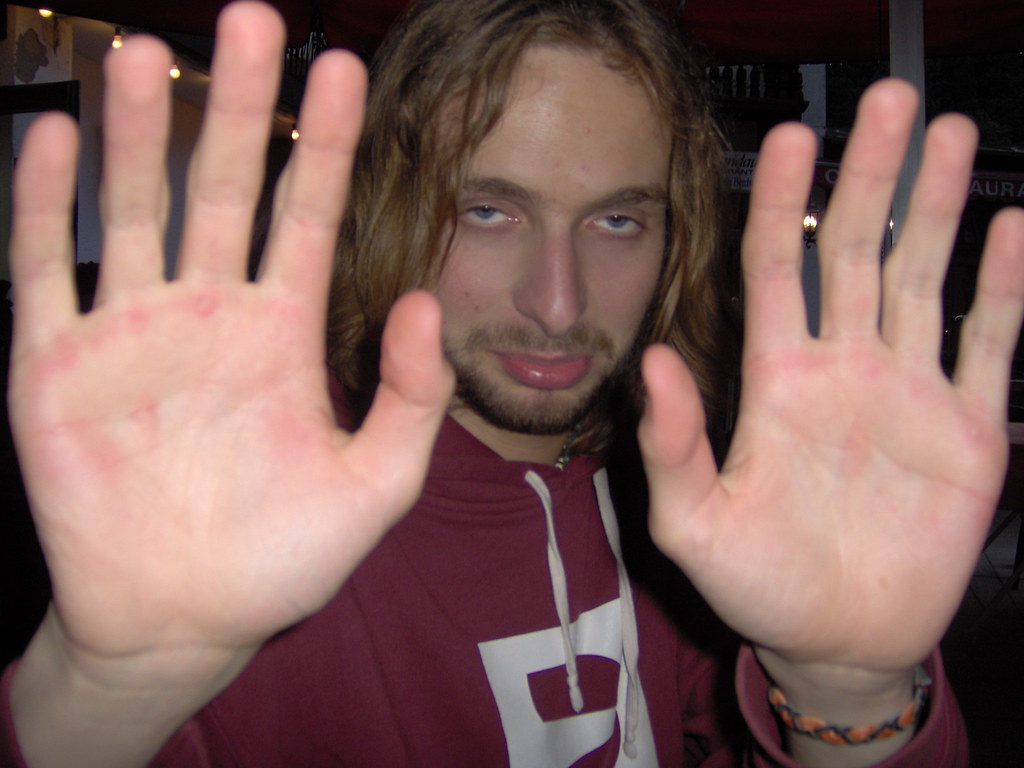A close-up photograph captures a young man inside, framed from his chest to just above his head. The flash from the camera accentuates his features, rendering the background indistinguishable. He appears either sullen or inebriated, with a pouty, protruding lower lip and grayish-blue eyes partially obscured by his expression. His long, brown hair falls around his face, complemented by a mustache and a short beard, potentially a full goatee.

He is wearing a maroon or burgundy hooded sweatshirt adorned with a white logo and white drawstrings at the neck. His left wrist sports a distinctive bracelet with a zigzag pattern, primarily in orange and possibly green or blue. The man holds both hands up, palms facing the camera, fingers splayed as if signaling "stop." This gesture, combined with his facial expression, conveys a mood of reluctance or discomfort with having his photo taken. His hands appear slightly reddened, suggesting they might be pressed against an unseen surface, possibly glass.